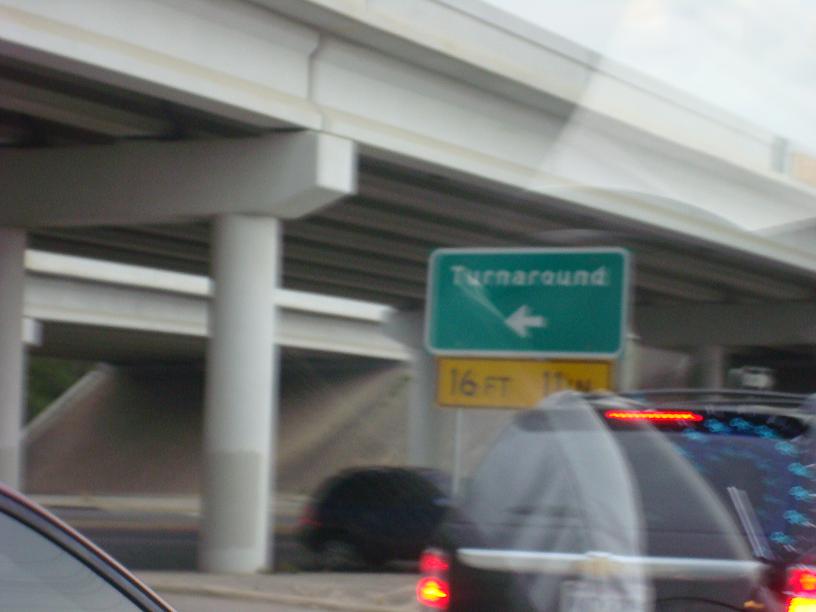A photo taken from the passenger seat of a moving car, driving under a double overpass bridge supported by tall concrete stilts. Approaching a T-intersection, a classic green rectangular road sign with white text and a left arrow instructs to "turn around." Below it, a yellow warning sign with a black border indicates the bridge clearance is 16 feet 11 inches. A black Chevy SUV with brake lights on is visible ahead, and another car is seen crossing the bridge perpendicularly. The scene is framed by a slightly cloudy sky, viewed through the car's windshield.